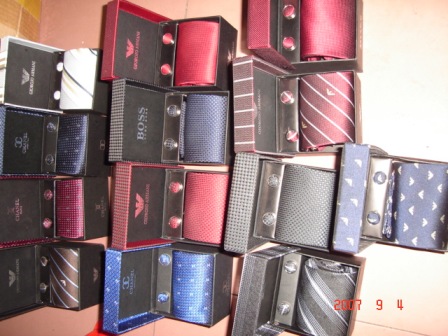This photograph, taken on a reddish-brown floor with the timestamp "2007-9-4" in red text at the bottom left corner, showcases a meticulously arranged set of men's neckties and cufflinks presented in designer boxes. The image captures 13 cube-like boxes, each open to reveal a rolled-up tie and two matching cufflinks. The ties are from various prestigious designers, including Hugo Boss, Armani, and Chanel, among others, which can be identified by the logos visible inside the opened boxes.

The ties display a vivid array of colors and patterns, with some featuring solid hues while others boast intricate designs. Among the collection, there are multiple shades of blue with white dotted patterns, deep metallic reds, and striped variations in brown and gray. A notable standout is a singular white tie with black stripes.

The boxes themselves are thoughtfully designed to complement the ties they hold, featuring matching or coordinated patterns and colors. For example, a tie with a blue background and white triangles is presented in a similarly patterned box with blue cufflinks, while another box presents a gray, black, and white striped tie with matching gray cufflinks. This careful attention to detail underscores the luxurious and cohesive nature of the display. The overall presentation, viewed from above, offers an appealingly detailed and organized glimpse into an exquisite collection of designer men's accessories.